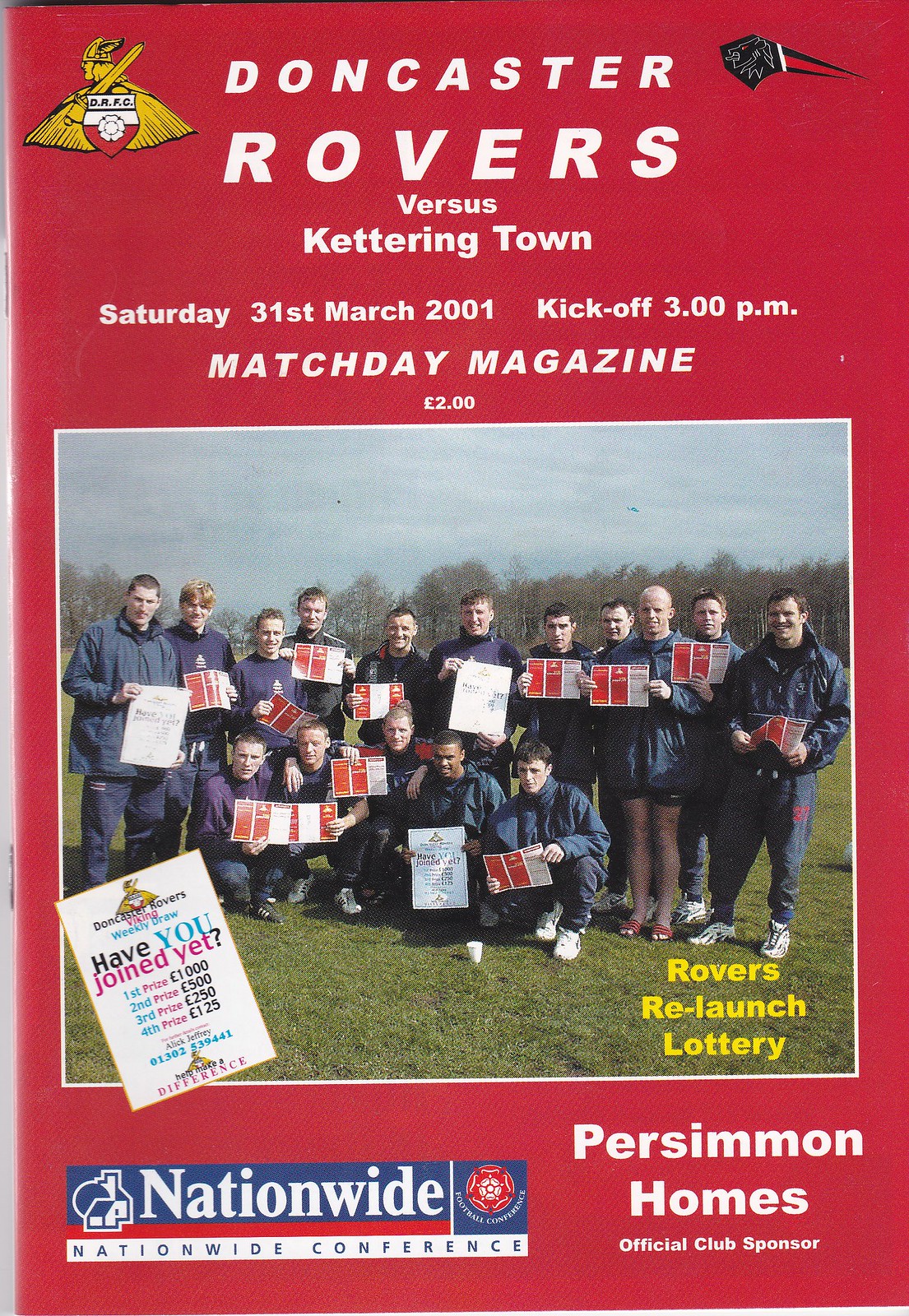The front cover of this vertically oriented Match Day magazine is predominantly red with white lettering. The magazine is for the soccer match between Doncaster Rovers and Kettering Town, scheduled for Saturday, 31st March 2001, with a 3 p.m. kick-off. Priced at £2, the cover features the Doncaster Rovers emblem on the left, which includes a Viking with wings holding a sword over a red and white shield. On the opposite side, the Kettering Town logo, resembling a black rock with streaks, is visible. 

Below these details, the centerpiece of the cover is a photograph taken outdoors, showing green grass and trees under a bluish-gray sky. The photo features a group of teenage boys, the team, some standing and others kneeling, all dressed in blue jackets and pants, though one wears shorts. They are holding red and white papers and are smiling. Overlaying the image are promotional texts such as "Rovers Relaunch Lottery" and "Doncaster Rovers Viking Weekly Draw: Have you joined yet? First prize £1,000, second prize £500, third prize £250, fourth prize £125." The magazine cover also notes the sponsorship from Nationwide Conference and Persimmon Homes at the bottom.